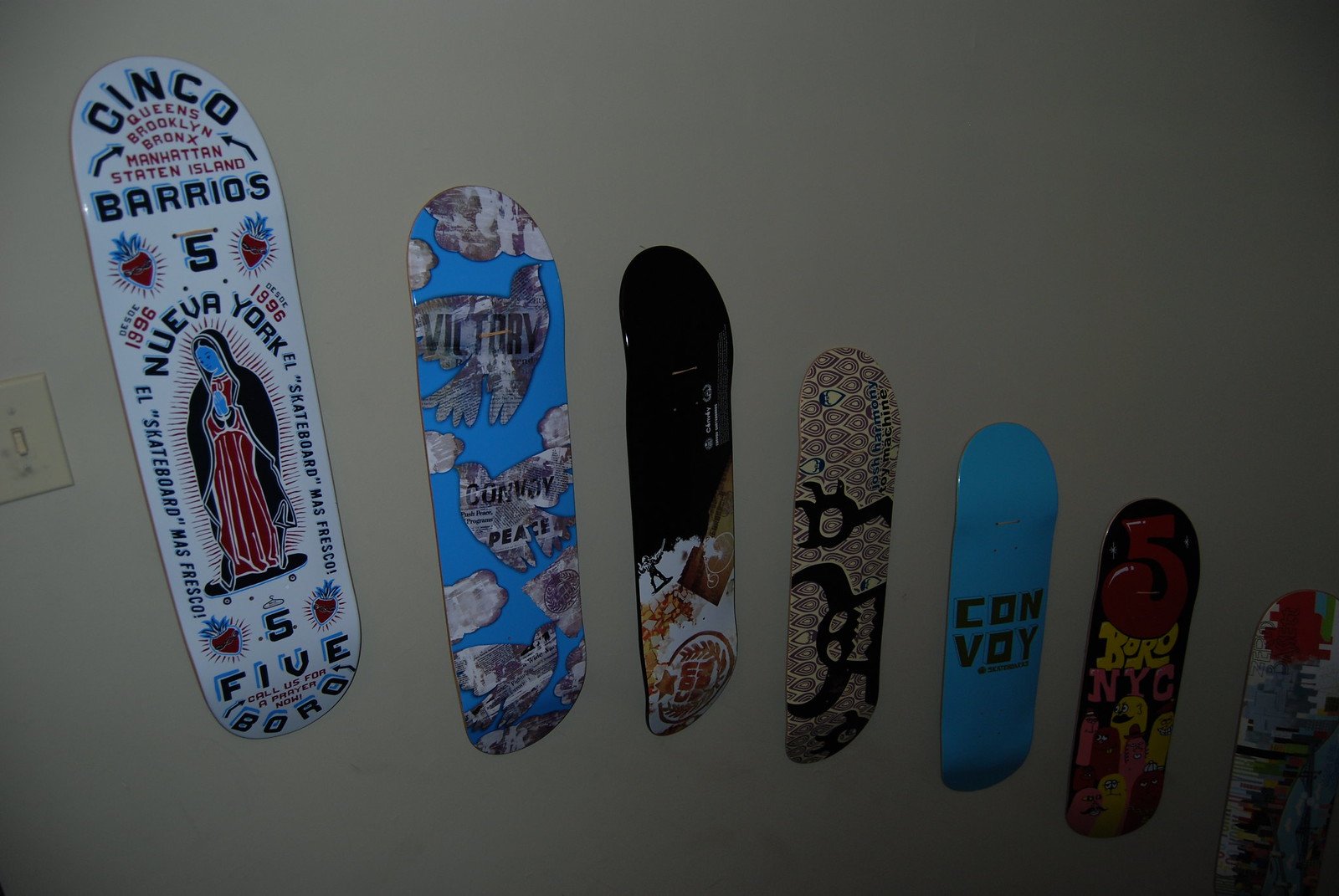In this dimly lit photo, a series of seven skateboard decks are mounted diagonally on a dark, possibly white-painted wall, making the details a little hard to see. On the far left, there's a light switch turned off. Each deck features distinct designs and vibrant colors. The deck on the far left is white and showcases an image of the Virgin Mary. To its right, another deck features the words "Cinco Barrios," listing New York City's five boroughs—Queens, Brooklyn, Bronx, Manhattan, and Staten Island—with a central design of the Statue of Liberty. Following that is a light blue deck with "Convoy" written in black text. The next deck is divided into half black and half white, followed by a gray one with a bubbled pattern and black outlines. The second to last deck is red with "Boro NYC" text, underlined by yellow and pink elements. The final deck on the far right is colorful but somewhat blurry, making the pattern indistinct. All these boards are arranged in a descending pattern from top to bottom, with each skateboard one inch lower than the previous one.